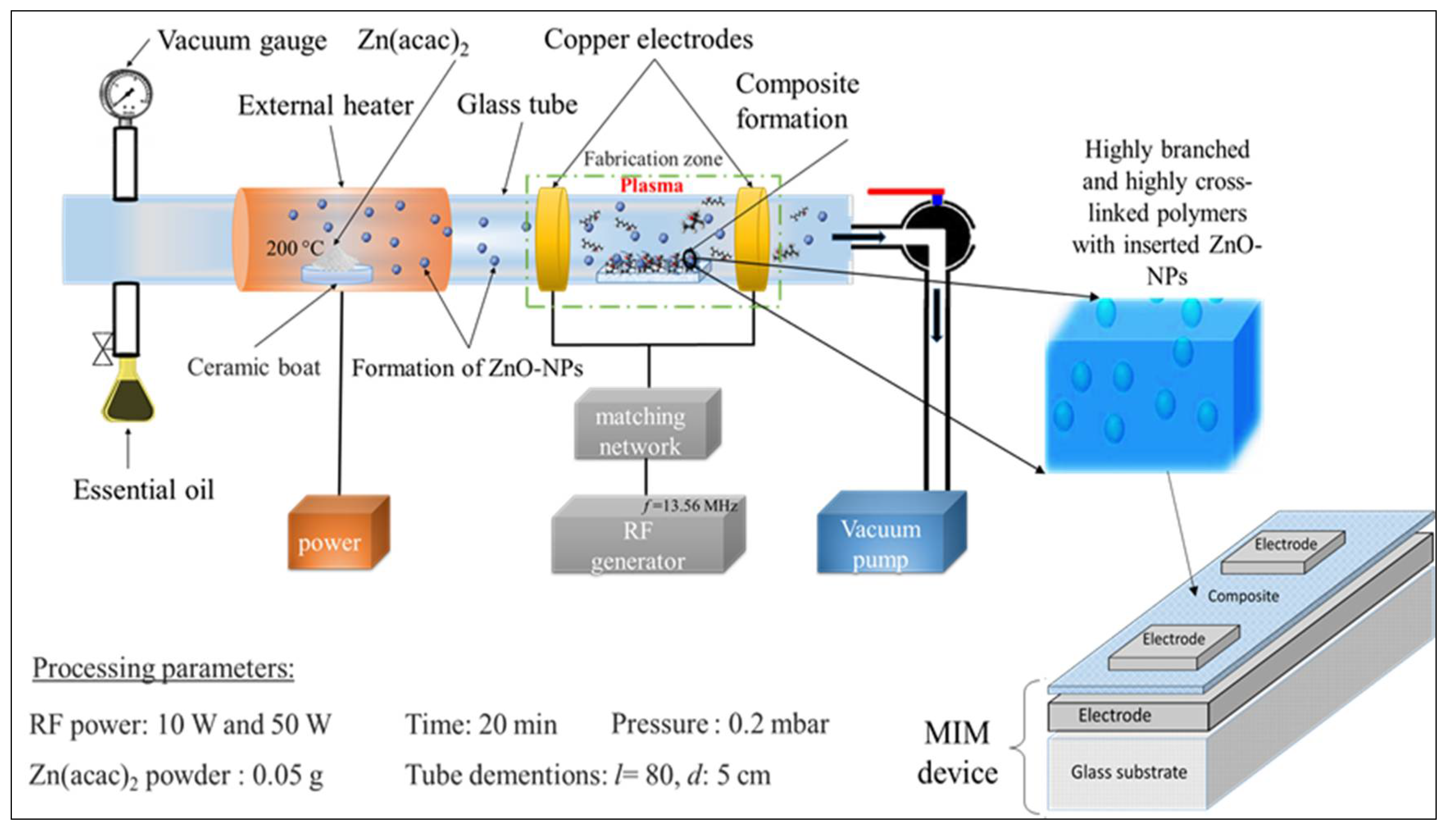The image is a detailed scientific diagram on a white background, enclosed in a thin black border typical of textbook illustrations. At the top left is a black circular gauge labeled "vacuum gauge ZN ACAC" attached to a vertical rectangle. Next to this is a pink horizontal rectangle marked "external heater 200 degrees Celsius," containing blue dots labeled "ZN ACAC2," denoting particles inside an orange section of a tube. The elongated blue horizontal rectangle represents a "glass tube," flanked by yellow rings labeled "copper electrodes" and black dots indicating "composite formation."

Adjacent to the glass tube, there’s a blue square with lighter blue dots that illustrate "highly branched and highly cross-linked polymers with inserted ZNO-NPs." Below the tube, schematic symbols for various devices and components are seen, such as an "RF generator" and a "vacuum pump," connected by lines and labels demonstrating components like "ceramic boat formation of ZNO-NPS" and "essential oil power matching network."

At the bottom of the diagram, detailed "processing parameters" are listed, including "RF power 10 watts and 50 watts," "time 20 minutes," "pressure 0.2 mbar," and "tube dimensions L = 80 cm, D 5 cm." The descriptive labels map out various interconnected parts like "MIM device" and "fabrication zone," forming a comprehensive visual guide of the scientific process being depicted.